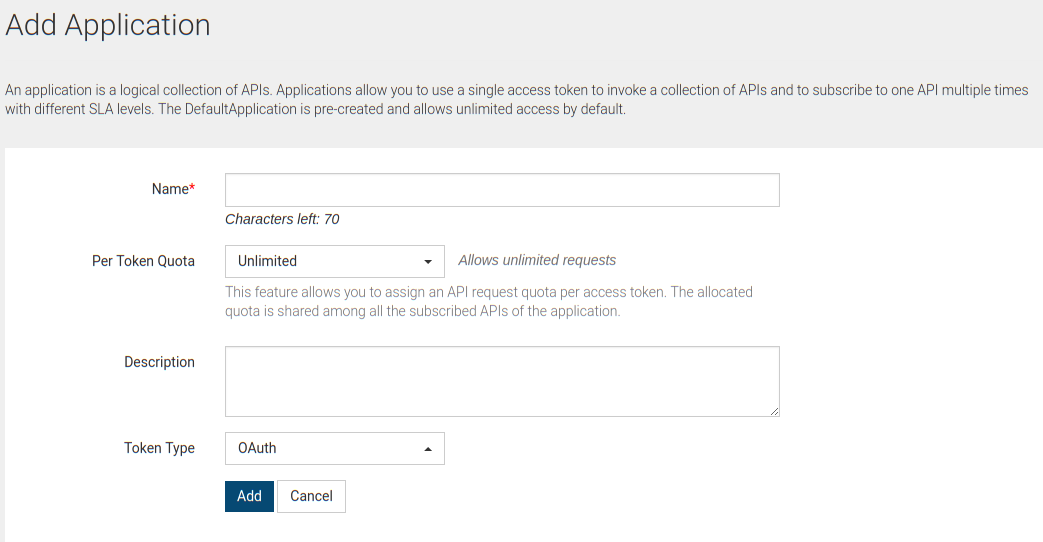**Caption: Detailed Screenshot of an Application Setup Interface**

The screenshot captures the setup interface of an application within a software platform. At the top, highlighted in grey, is the heading "Add Application." This section serves as a brief explanation of what an application constitutes—a logical collection of APIs. The instructions further explain that applications enable the use of a single access token to invoke multiple APIs and allow for multiple subscriptions to a single API with varying SLA levels. The default application, which is pre-created, provides unlimited access as a standard feature.

Below the heading, the user interface transitions to a light-grey rectangular section, followed by a completely white background area. Here, users find a text box titled "Name," with a character limit of 70, as indicated by the message "Characters left: 70" beneath the text box.

Moving further down, there is a label "Per Token Quota" accompanied by a dropdown menu set to "Unlimited," allowing for unlimited requests. An explanatory note follows, clarifying that this feature assigns an API request quota per access token and that the allocated quota is shared among all the subscribed APIs of the application.

Below this, a section labeled "Description" features a blank text box for additional details. Further down, there's another dropdown menu under "Token Type," currently set to "OAuth."

The interface concludes with two buttons at the bottom: a blue "Add" button for saving the application setup and a white "Cancel" button for aborting the process.

This well-structured interface is designed to streamline the process of configuring applications, emphasizing clarity and user-friendliness.